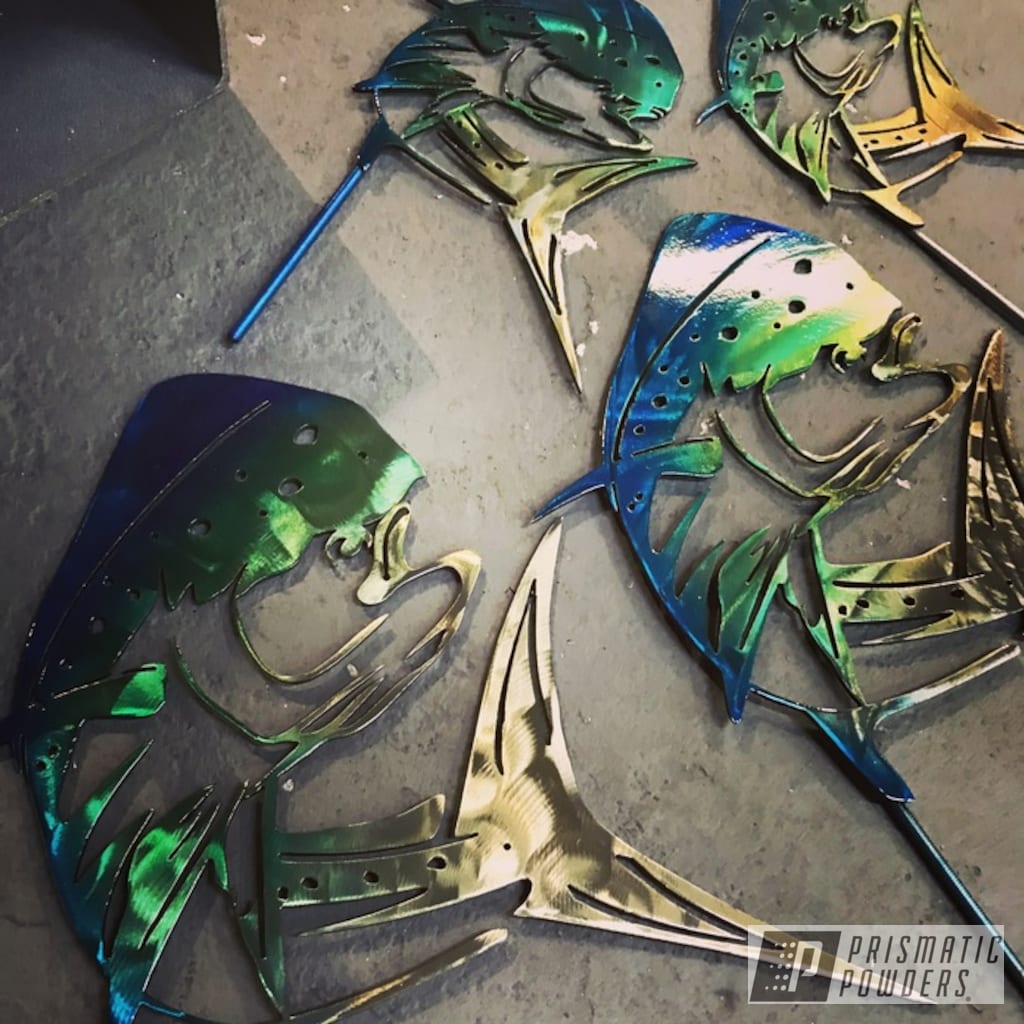The photograph showcases an array of artful metal objects that resemble fish or possibly sharks, laid out on a brown, perhaps dirty concrete floor, which might be a garage floor. These elaborate designs feature a stunning, oil-slick finish that transitions from a shiny blue to green and yellow, evoking the iridescent quality of a rainbow. Each fish-like object has fins and tapers into a pointed bottom, with blue metallic rods extending from their bases, suggesting they might be signs or decorative pieces. Notably, in the bottom right corner of the image, there is an inscription of "Prismatic Powders" in white outlined and gray lettering, adding a touch of branding to the artwork. The composition is harmonious yet complex, with each piece reflecting light in a way that emphasizes their intricate, multi-colored metallic sheen. The scattered arrangement also includes additional similar fish-like objects on the top right, all enhancing the visual appeal and adding layers of depth to the scene.